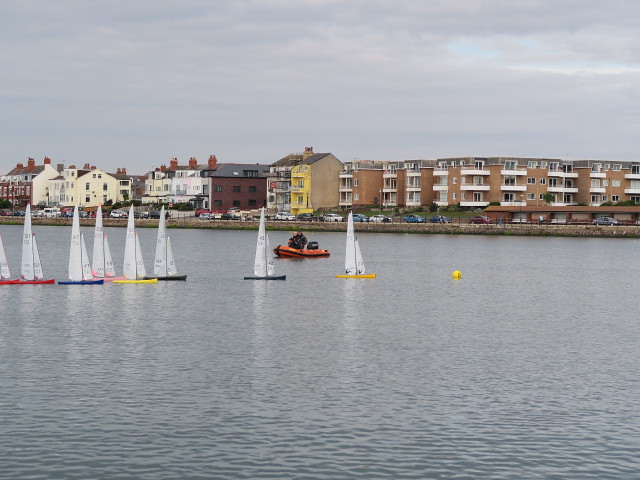This photograph captures a scene of a river adorned with a variety of colorful sailboats set against the backdrop of an English-style coastal cityscape. Dominating the lower half of the image, the river features seven model sailboats, clustered mainly on the left side, with red, blue, pink, yellow, and black sails jutting out in triangular forms. A conspicuous yellow buoy marks the water, and in the background, an orange raft with people provides a sense of scale, demonstrating the miniature size of the sailboats. 

The middle portion of the image vividly depicts an array of apartment buildings stretching from left to right. On the left, the structures appear box-like with small roofs, characterized by rows of windows. Central to the photo and extending to the right, the architecture transitions to a more stately design, consisting predominantly of flat-topped, brick buildings punctuated by white-trimmed windows and balconies jutting out from double glass doors. Interspersed among these buildings is a striking bright yellow structure with a black roof, standing out against the brick façades. 

Above, a dark gray sky unfurls across the top of the image, with sporadic streaks of light blue breaking through the clouds in the top right corner, hinting at a patch of clearer weather. The city's edge is marked by a light brown concrete wall, just beneath a line of parked cars visible to the far right. This intricate layering of river, city, and sky combines to create a detailed and dynamic composition.